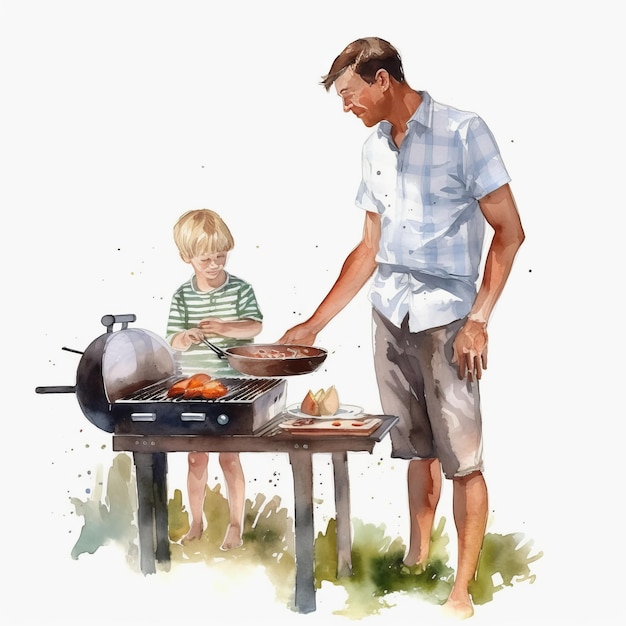In what appears to be a watercolor painting set against an off-white background tinged with gray, a man and a young boy are engaged in a leisurely outdoor cooking session. The man, with dark brown hair and slightly tanned skin, is clad in a short-sleeved, collared shirt with a plaid pattern and knee-length shorts. To his right stands a small boy with blond hair, donned in a green and white striped shirt. They stand over a small grill placed on a table, its lid open to reveal various foods cooking, including a very large pan. The man, holding a pan in his right hand, appears to be lifting it off the grill as he smiles down at it. The boy, looking intently at the pan, seems fascinated by the cooking process. The table also bears a plate filled with teardrop-shaped items and various cooking utensils. Their feet rest on a patch of grass, with dots scattered around them that might represent flies or simply add texture to the scene, juxtaposed against the largely plain background.